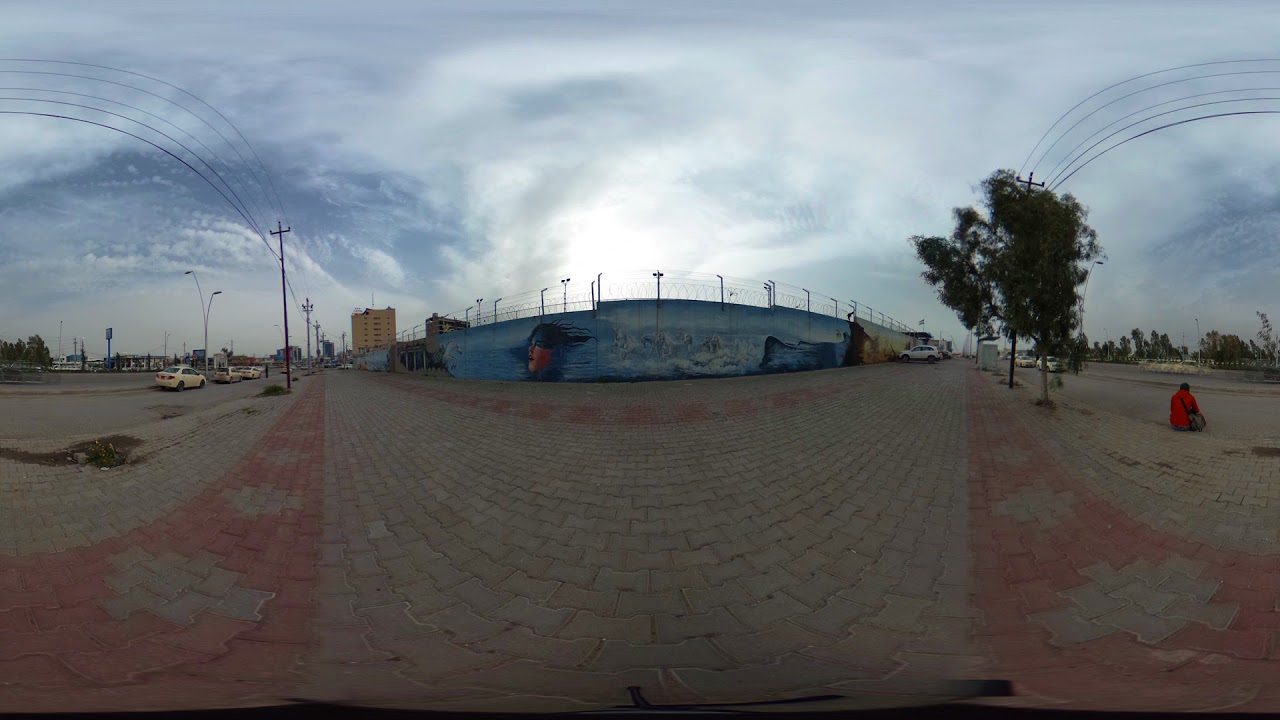The photo captures an overcast urban environment, seemingly taken with a 360-degree or wide-angle lens that causes the image to appear warped and distorted, especially around the edges. Dominating the left side of the image is a street with power lines that curve oddly forward, likely a result of the panoramic technique used. This street is lined with several white cars and features buildings further down in the distance. Centrally, a tall concrete wall decorated with vibrant murals, including one of a smiling woman with wind-swept hair standing before an ocean, extends almost to the right side of the image. The wall is topped with barbed wire and has a cobblestone pathway in front of it. Near the right side of the wall, a car is parked, leading to a sidewalk flanked by numerous trees. Beyond the sidewalk is another street with more cars of various colors, largely beige or yellow, and more curved telephone wires. A person in a red shirt, possibly carrying a bag, sits by the curb. Background elements include some stadium lighting and distant city buildings. The entire scene is set under a grayish-blue, cloudy sky, suggesting it may rain.